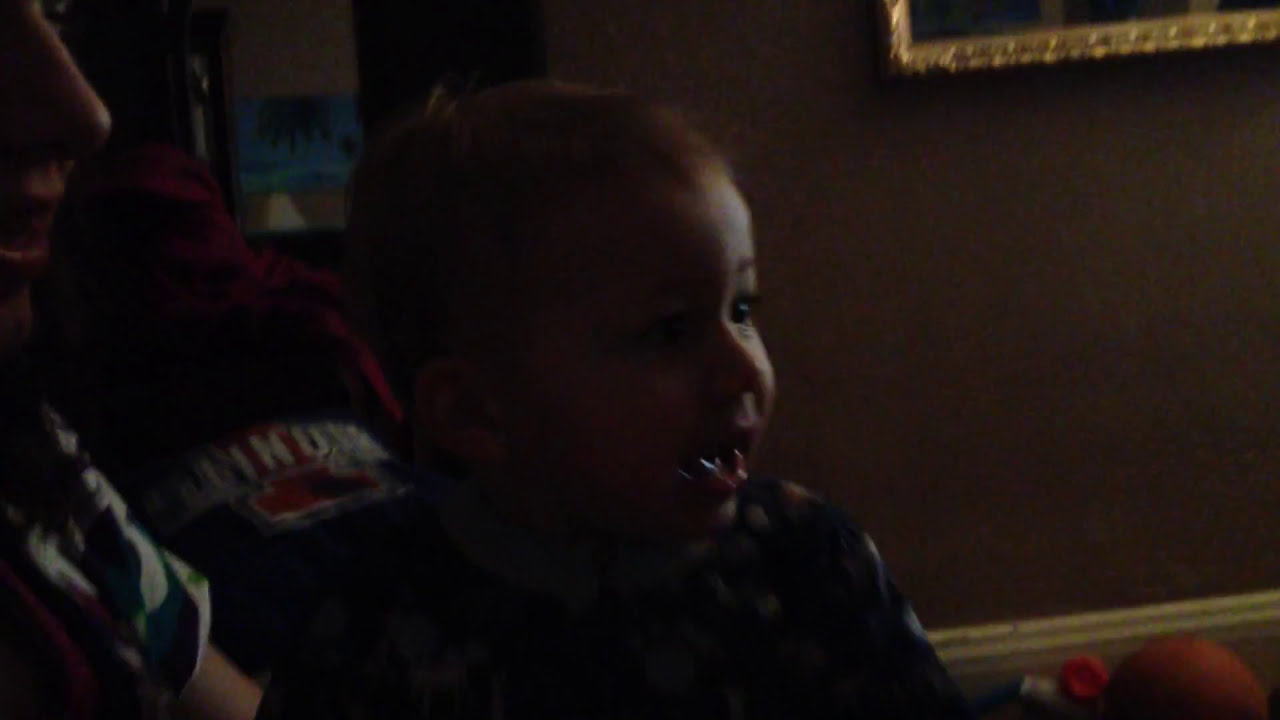In a dimly lit room, this evocative photograph captures a young toddler who looks to be around two years old. The setting appears to be nighttime indoors, possibly with a soft light source illuminating from the right side of the image. The child's face is predominantly in shadow except for a portion on the left, revealing their delicate and youthful features. Light wispy hair and a high-collared outfit frame their excited expression, with their mouth slightly open and eyes looking towards the right. The composition centers the child within the horizontal rectangle of the photograph, showing them from the chest up. 

A woman's face and upper body are partially visible to the left, from the top of her head down to her arm, indicating she may be holding the toddler. The dark, underexposed background faintly reveals additional elements: a beige wall, a gold-framed picture in the upper right corner, and some white molding near the floor. Colors in the image range across gold, brown, white, red, burgundy, beige, black, and gray, contributing to the warm, homey ambiance of the setting.